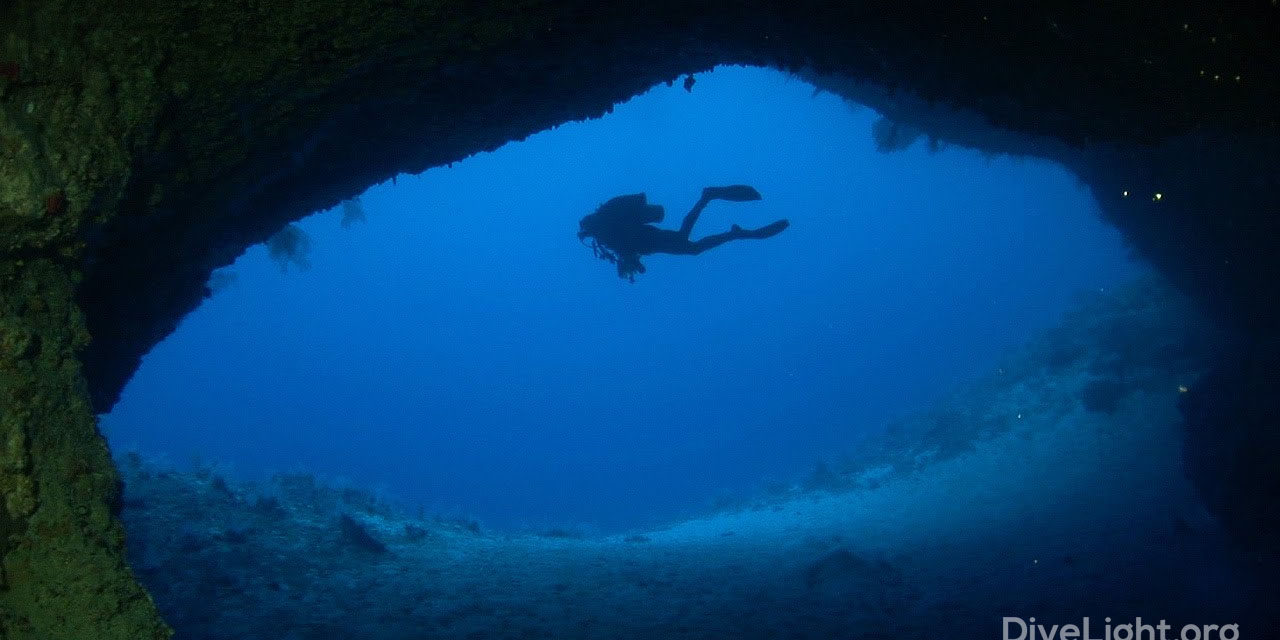In this horizontal underwater photograph, a scuba diver is seen in silhouette at the mouth of a dark, underwater cave or tunnel, facing left. The diver is equipped with flippers and an oxygen tank, and their profile is framed by the cave's entrance. The walls of the cave are coated with green algae or sea moss, giving a fuzzy appearance to some of the rocks. The surrounding ocean is a vibrant blue, with a gradient that transitions from lighter blue at the top to darker blue at the bottom. The seafloor, which appears sandy, arcs upward mostly to the right and features some scattered ocean debris. In the upper right of the image, several pale yellow dots—potentially light artifacts or bioluminescent creatures—are noticeable, with two distinct yellow dots also present. The white text "divelight.org" appears in the bottom right corner of the image, indicating the probable source or host of the photograph.